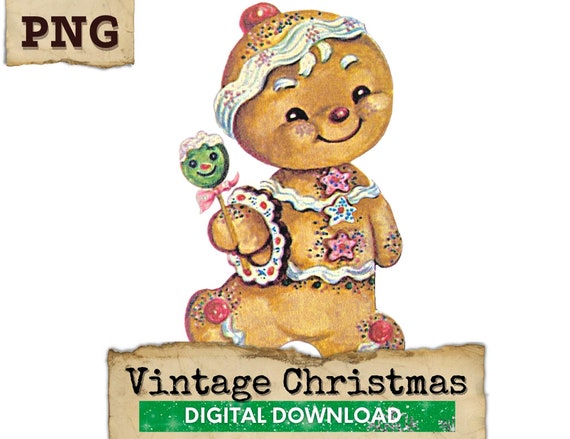The image depicts a whimsical, vintage-style Christmas illustration labeled with "PNG" in the top left corner and "Vintage Christmas Digital Downloads" at the bottom on a torn paper background. The centerpiece is a cartoon gingerbread man, prominently smiling with two black beady eyes and eyebrows made of icing. This festive figure wears an icing adornment that resembles a headband, with a cherry-like candy bead poised atop its head resembling a Christmas hat, and sprinkles scattered across its body. The gingerbread man is decorated with star-shaped buttons along its chest, sprinkled and icing-laden, and is adorned with intricate frosting details: a waistband, and a necklace. It's captured in a dynamic pose, seemingly mid-walk, with a green, smiley-face lollipop held in its right hand. The entire scene evokes a cheery, nostalgic holiday spirit.